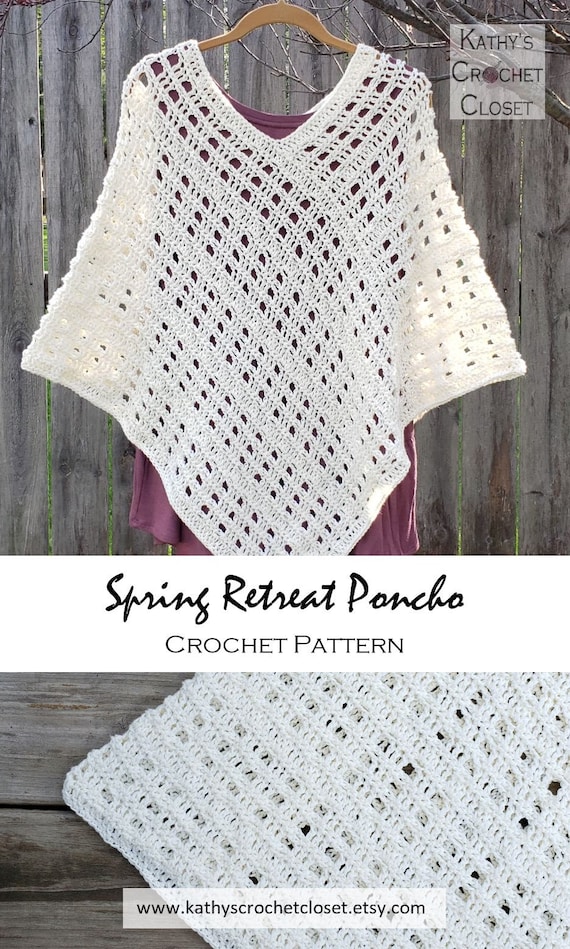The image is an advertising poster for an Etsy shop named Kathy's Crochet Closet, promoting a handcrafted white crochet poncho named "Spring Retreat Poncho." The poster contains two photos: the top photo displays the entire poncho, elegantly hanging on a wooden hanger over a pink t-shirt, set against the backdrop of an old wooden fence, with large, intricate openings in the crochet work. The top right corner features the shop's logo, "Kathy's Crochet Closet," in black text on a white background. The central part of the poster prominently highlights the name of the crochet pattern, "Spring Retreat Poncho," in cursive, followed by the words "Crochet Pattern" in plain font. The bottom photo offers a close-up view of the detailed crochet material, along with the shop's URL, www.kathyscrochetcloset.etsy.com, centered and in black font.